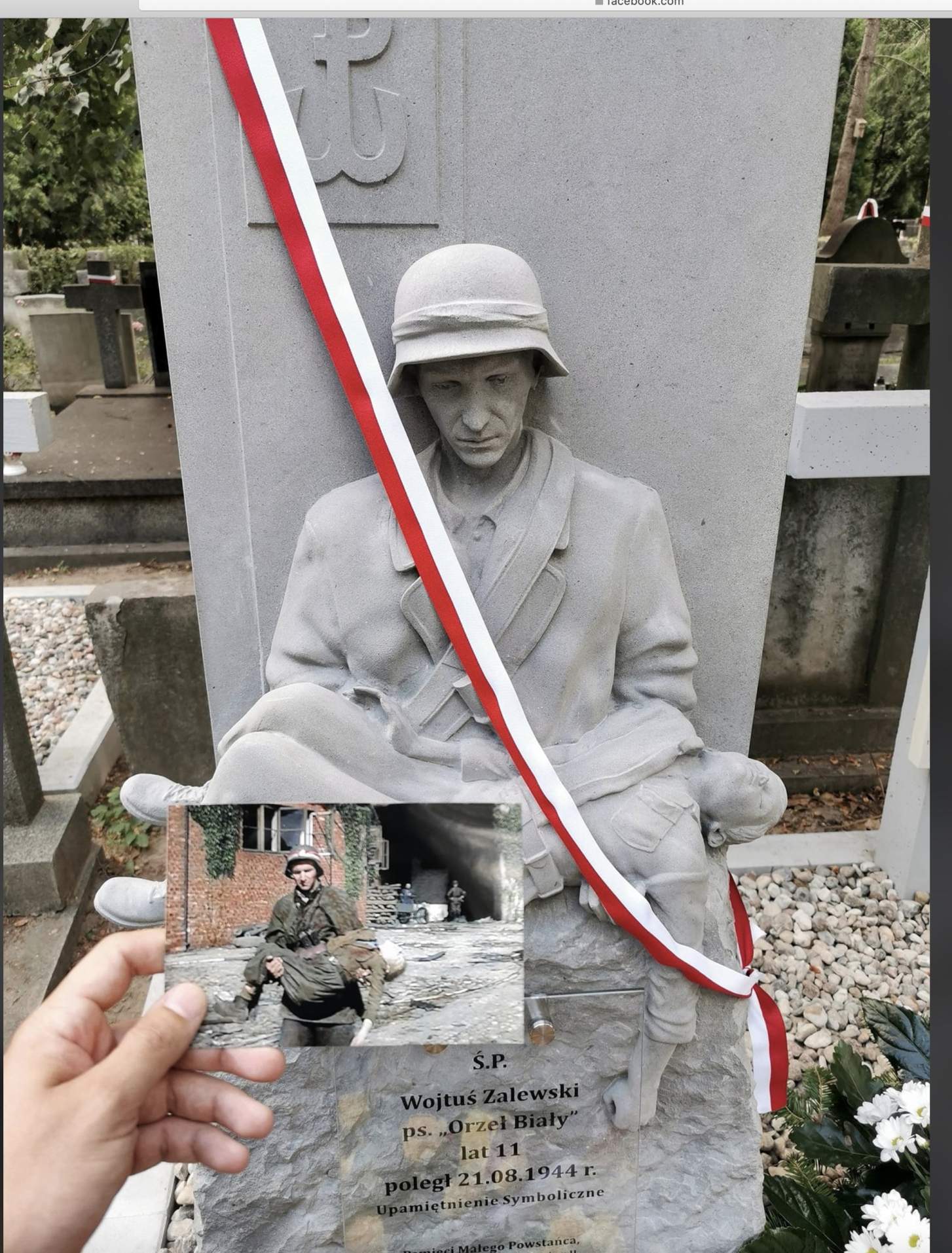In this vertical rectangular image, a profound and somber scene is depicted at a cemetery. Central to the image is a light gray statue of a military soldier sitting on the ground, exuding sadness as he looks down. The soldier, adorned in a coat and helmet, cradles another soldier in his arms. The base of the statue serves as a grave marker, inscribed with the name "Wojtus Zalewski," with details of his life.

In front of the statue, emerging from the lower left corner, a hand holds a photograph that mirrors the statue’s scene—a soldier in uniform carrying another person out of a building. Surrounding the grave marker are white and gray rocks within a flowerbed, which also holds some white flowers to the right of the statue. Crosses and additional grave markers are visible in the background, enhancing the solemn ambiance of the cemetery.